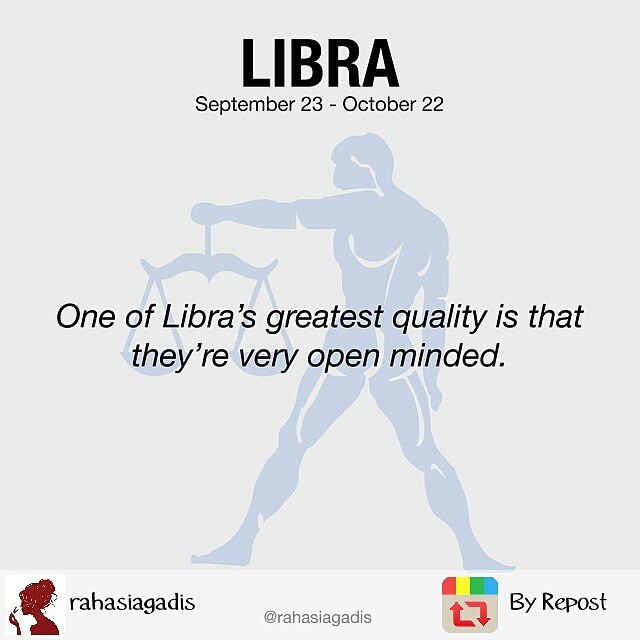The image is a social media post with a gray background and a promotional feel. At the top, the text "LIBRA" in bold black letters announces the zodiac sign, followed by the dates "September 23rd to October 22nd," where only the 'S' and 'O' are capitalized. Dominating the center of the image is a blue graphic of a naked man holding a pair of scales, symbolizing Libra. Below this graphic, black text reads, "One of Libra's greatest quality is that they're very open-minded."

In the bottom left corner, there's a square image of a red profile of a woman with a beehive hairdo, adjacent to the name "RAHASAGADIS" in black font. The bottom right corner features a logo with two arrows and a rainbow-colored tab, accompanied by the text "BUY REPOST." The overall aesthetic combines a blend of blue tones for the central figure and a red accent, reinforcing the artistic and astrological theme.